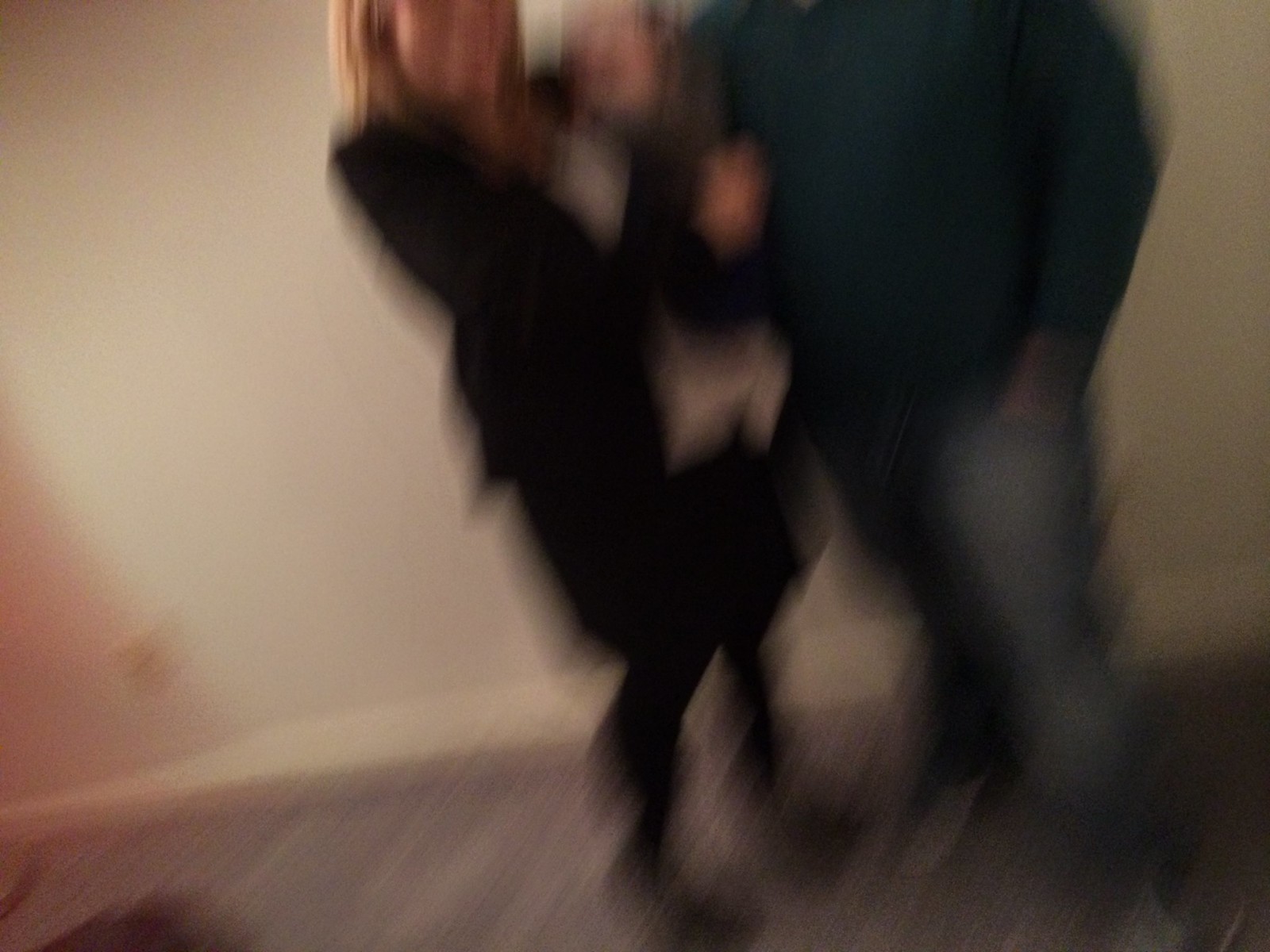In the image provided, a blurry depiction of a small family can be observed. Positioned to the right side of the image, the family consists of three individuals: a woman, a man, and their child. The woman's face is faintly visible; she has blonde hair and is dressed in a black suit, which appears to include black tights. The man, whose face is partially cut off at the shoulder, is wearing a blue dress shirt paired with jeans and has his hand in his pocket. The child, a baby, is being held, but like the woman, its face is barely discernible due to the blurriness.

They are standing in a hallway with a blue carpet underfoot. The background comprises a white wall with a white baseboard and a visible electrical outlet, adding detail to the setting. Despite the image’s lack of clarity, the familial bond and casual demeanor of the subjects are evident.